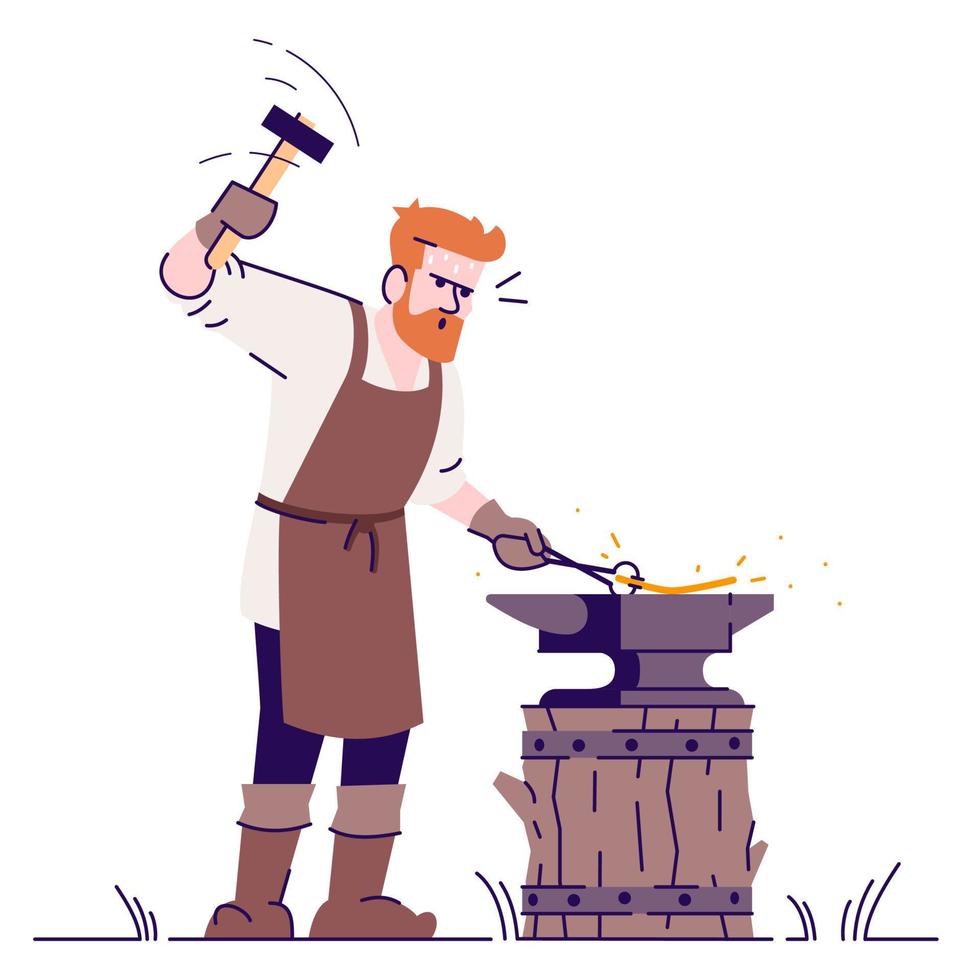This illustration is a vibrant, cartoon-like depiction of a determined blacksmith at work. Positioned to the left of the image, the male blacksmith is facing to the right, his orange hair and full beard contrasting sharply with his white long-sleeve shirt. He is clad in a brown protective apron, brown gloves, denim pants, and knee-high brown boots. The blacksmith's face is covered in sweat, emphasizing his hard labor. He is holding a metal hammer in his raised right hand, with motion lines indicating the imminent strike. In his left hand, he grasps a pair of tongs, securing a yellow, white-hot piece of metal atop a sturdy brown anvil, which rests on a wooden stump. Sparks fly as he prepares to hammer the glowing metal, capturing the dynamic and intense nature of his craft in this animated scene.